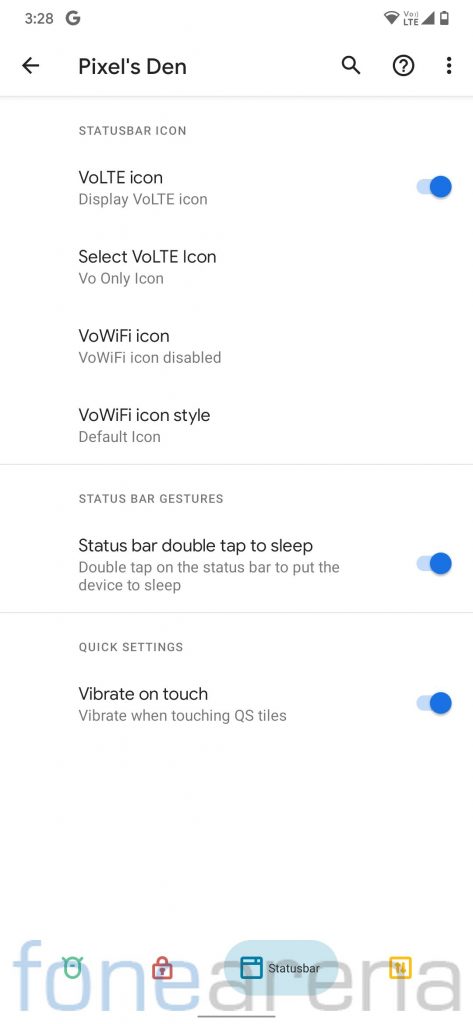Edited screenshot of a Google Pixel settings screen. The top left shows "Pixel's Thin" in bold black letters, accompanied by a back arrow leading to the previous settings menu. To the right, there are icons for search (magnifying glass), help (question mark), and the menu (three vertical dots). Below this header, a vertical array of categories and subcategories is displayed. 

At the very top, there is a status bar icon with small grey letters. Below it, the "VoLTE icon" option is mentioned in small black letters, with an accompanying label "Display VoLTE icon" and a toggle switch set to on. Further down, the option "Select VoLTE icon" is followed by "VoOnly icon," "VoWiFi icon" (which is disabled), and "default icon."
  
Next, under the status category "Status Bar," written in small grey font, the option for "Status Bar Double Tap to Sleep" (toggled on) is present. Then, under "Quick Settings," the "Vibrate on Touch" option is also toggled on.
  
The screenshot ends with a watermark from Phone Arena at the bottom.